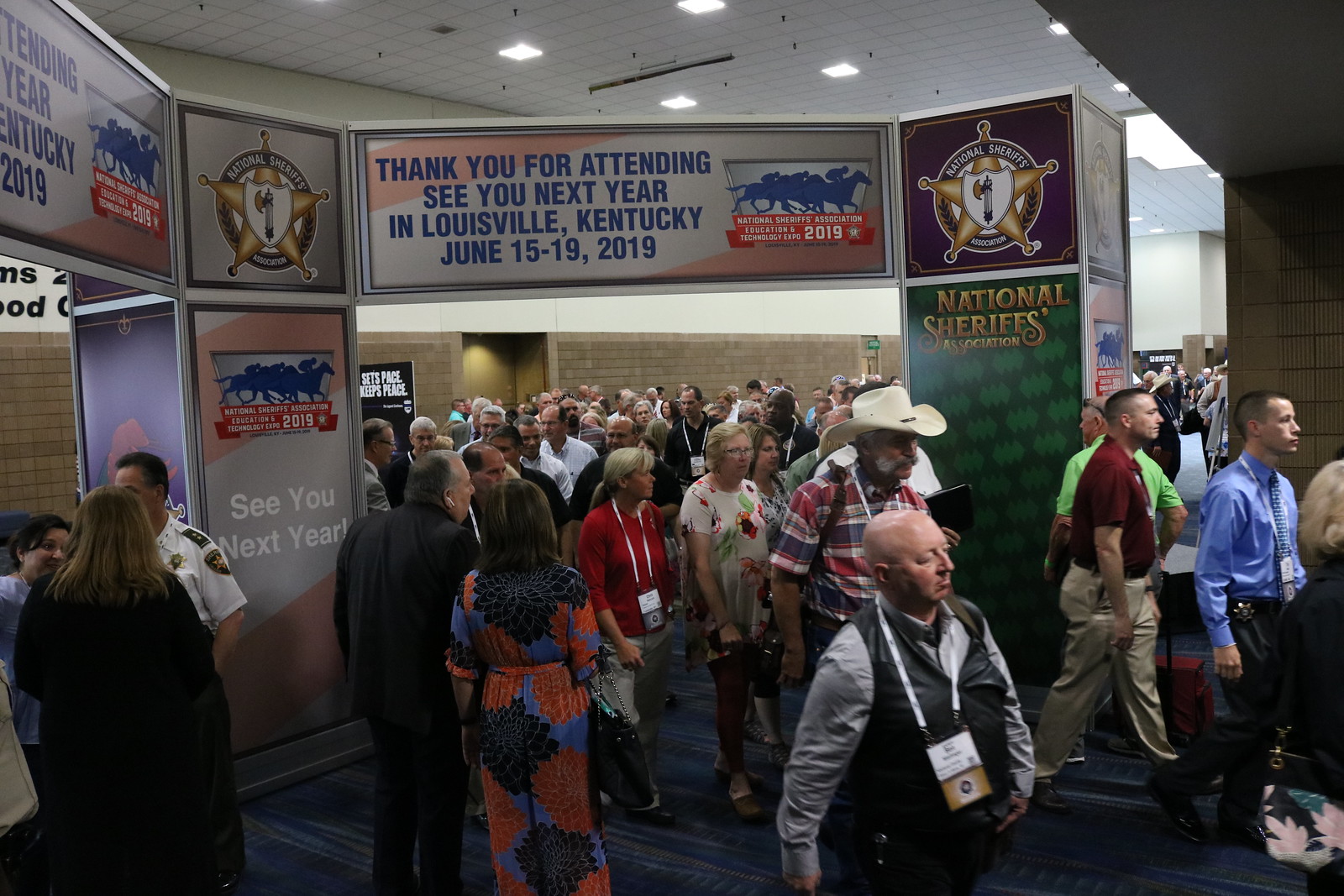The image captures a bustling scene at the National Sheriffs Association Education and Technology Expo 2019. In the foreground, a diverse crowd is walking on a blue and gray carpet, appearing tired and some looking disappointed, possibly indicating they might have faced losses or an exhaustive day. The attendees, who are primarily older and of a white background, are all wearing lanyards with name tags. A tall archway dominates the top of the image, emblazoned with a sign in bold blue letters that reads, "Thank you for attending. See you next year in Louisville, Kentucky, June 15th through 19th, 2019." Adjacent to the arch is a logo depicting several horses shaded in blue and the event name, reinforcing the connection to Louisville, Kentucky. The white square-tiled ceiling with integrated lights provides a neutral backdrop to the scene, while on the periphery, a security guard stands vigilant, contributing to the organized yet bustling atmosphere of the event’s conclusion.